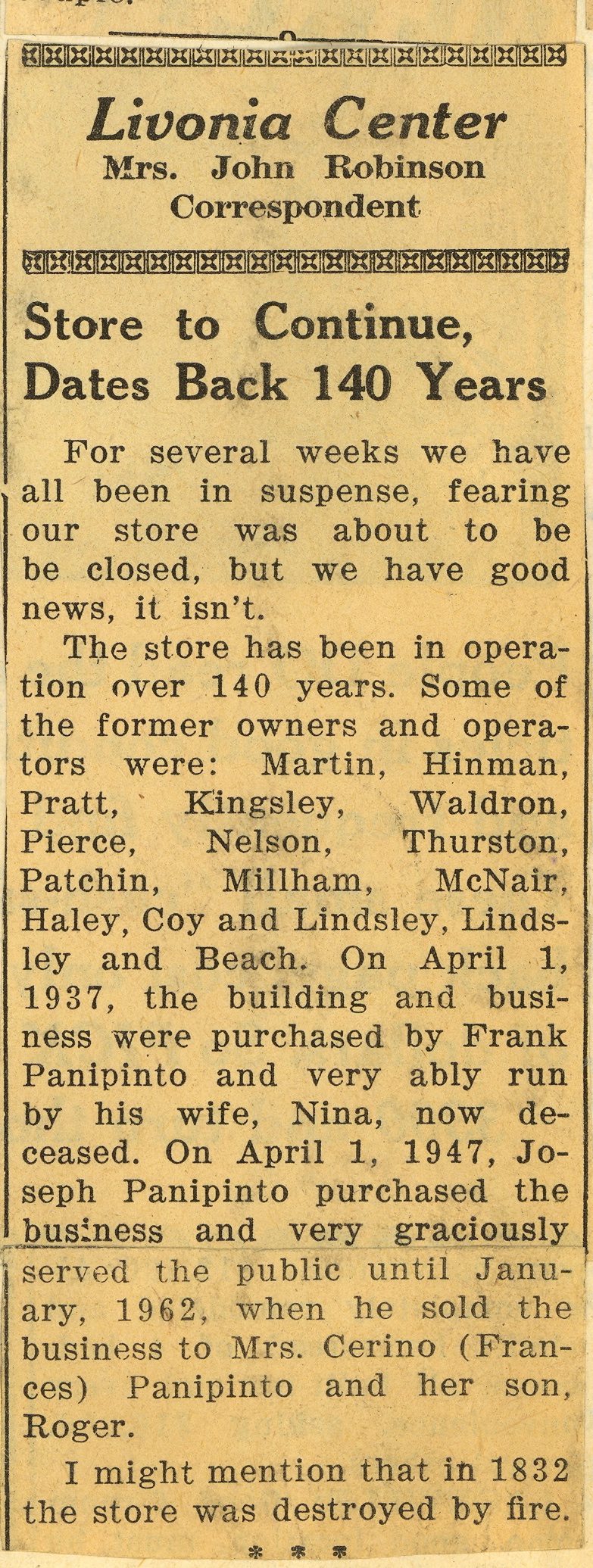The image is a highly faded, yellowed newspaper clipping from Livonia Center, scripted by Mrs. John Robinson as correspondent. The prominently featured column titled "Store to Continue" commemorates an establishment that has remarkably withstood the test of time, operating for over 140 years. The article recounts the anxious weeks during which the community feared the store’s imminent closure, only to be relieved by the announcement that it will remain open.

Detailing the store’s storied past, the article lists a succession of former owners and operators, including Martin, Hinman, Pratt, Kingsley, Waldron, Pierce, Nielsen, Thurston, Patchen, Millham, McNair, Haley, Coy, and the duo Linsley and Beach. A significant milestone in the store's history occurred on April 1, 1937, when Frank Panepinto acquired the building and business, which were adeptly managed by his late wife, Nina. Following this, on April 1, 1947, Joseph Panepinto took ownership and graciously served the public until January 1962, when the business was ultimately sold to Mrs. Serino. The clipping also touches upon a historical calamity when the store was destroyed by fire in 1832, underscoring its resilience and continuity over the decades.